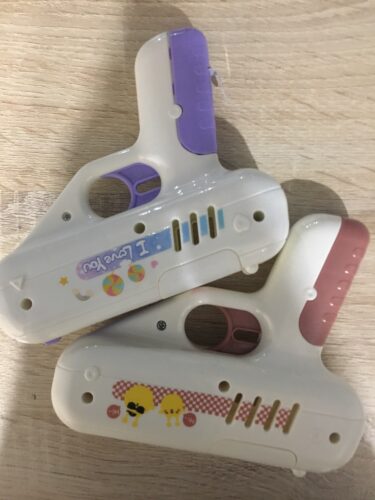In the image, two toy guns are laid out on a beige wooden surface with noticeable darker grains running horizontally across what appears to be a table or countertop. Both toy guns are placed upside down with their handles pointing upward. The gun at the top features a handle in purple and white, and it has additional purple detailing. The main body of this gun is decorated in shades of blue and white, with a prominent blue streak that reads "I love you" written upside down. Accompanying this phrase are two balloons in orange, blue, and yellow just below it.

The bottom gun mirrors the top one's design but is adorned in a different color scheme. This gun has a handle in dark pink and white, along with a dark pink trigger. Its central area includes a white and red checker pattern and is embellished with two yellow creatures on the left side, one of which appears to be wearing sunglasses. Both guns are made of plastic and present a playful, colorful aesthetic against the light brown wooden backdrop.